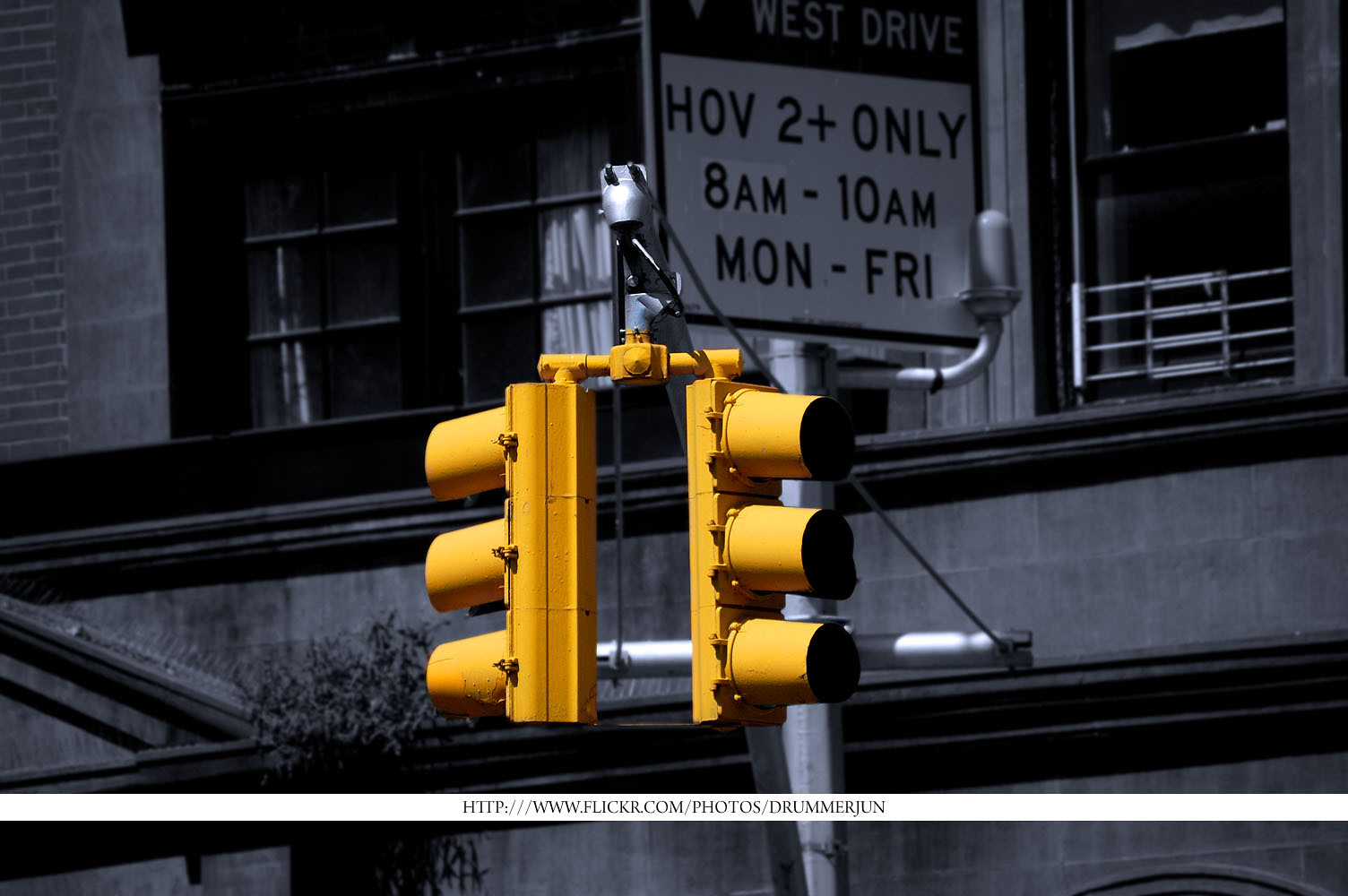This black-and-white photograph captures a quiet street, primarily monochrome, but highlighted by two vibrant yellow street lights and a set of traffic lights displaying four stacked signals in red, yellow, and green. Prominently featured is a street sign that reads, "West Drive, HOV 2+, Only 8am to 10am, Mon to Fri." In the background, a building with distinctive architectural features is visible, including a set of double doors adorned with curtains, adjacent to a window or stairwell framed with silver railings. The image also captures partial foliage from a nearby tree. The photograph credits are visible at the bottom, indicating it's sourced from www.flickr.com/photos/dramajune.